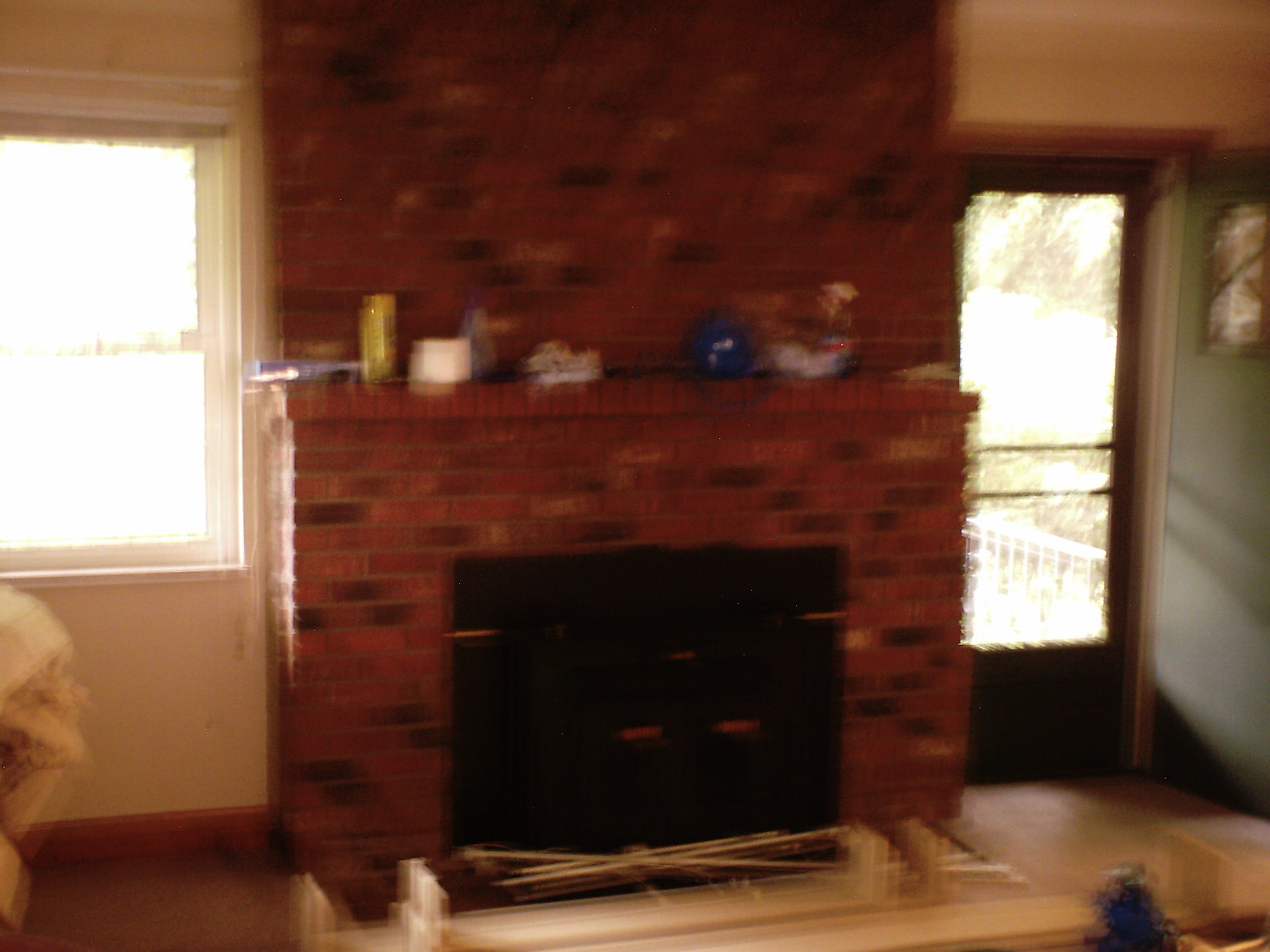In this somewhat blurry photograph of an interior scene, the focal point is a traditional red brick fireplace with a black grill cover that extends up to the ceiling, occupying the central portion of the image. The fireplace features a cluttered mantle with various items, including a recognizable bottle of Windex, a spray can possibly of Pledge, a blue circular object roughly the size of a bowling ball, and several other white containers. Beneath the fireplace, the floor is scattered with what seem to be crisscrossed materials and possibly benches or wooden pieces, suggesting that the area might be undergoing renovation. To the left of the fireplace, there is a window trimmed in white, which allows light to stream into the room. On the right, there’s a black door that opens to reveal a clear glass storm door, offering a serene view of the outdoors. The walls surrounding the fireplace are white with brown trim at the bottom, contributing to the overall traditional yet lived-in feel of the room.